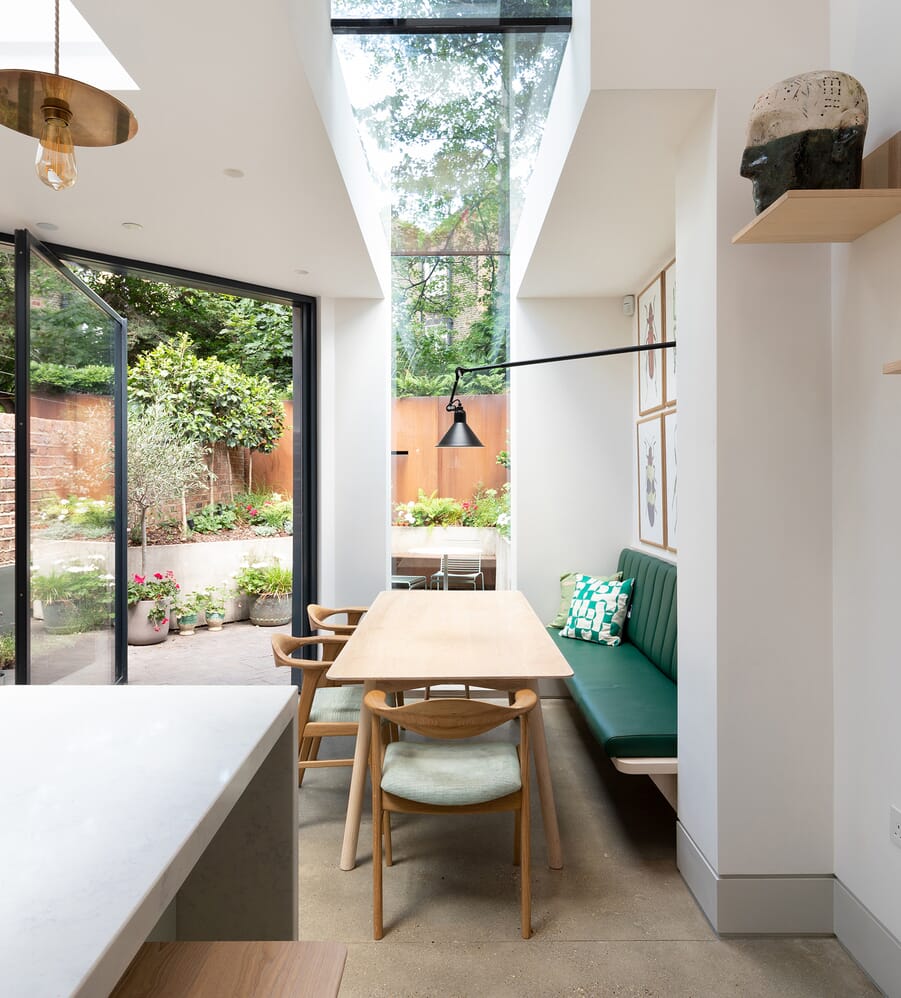The image depicts a sunlit dining area within a home, characterized by its narrow, hallway-like layout. On the left side, a long, foldable white countertop extends into the space, while the floor beneath is a textured brown concrete. Central to the room is a rectangular wooden table, surrounded by a mix of seating options: three cushioned wooden chairs and a green cushioned bench against the right wall, which features a decorative throw pillow. This bench has built-in storage or seating, reminiscent of a cozy restaurant booth. 

A sleek metal pole protruding from the wall supports a spotlight that casts a warm glow on the empty table below. Above the cushioned bench, a small wooden shelf holds a statue of a face, adding an artistic element to the otherwise minimalist decor. The walls throughout are crisp white, complemented by gray baseboards, and large black-framed windows on the left side flood the area with natural light, providing a clear view of the charming backyard. Outside, a wooden fence surrounds a garden filled with various potted plants and flowers. Notably, the ceiling above the table is made of glass, further enhancing the room's airy and open ambiance.